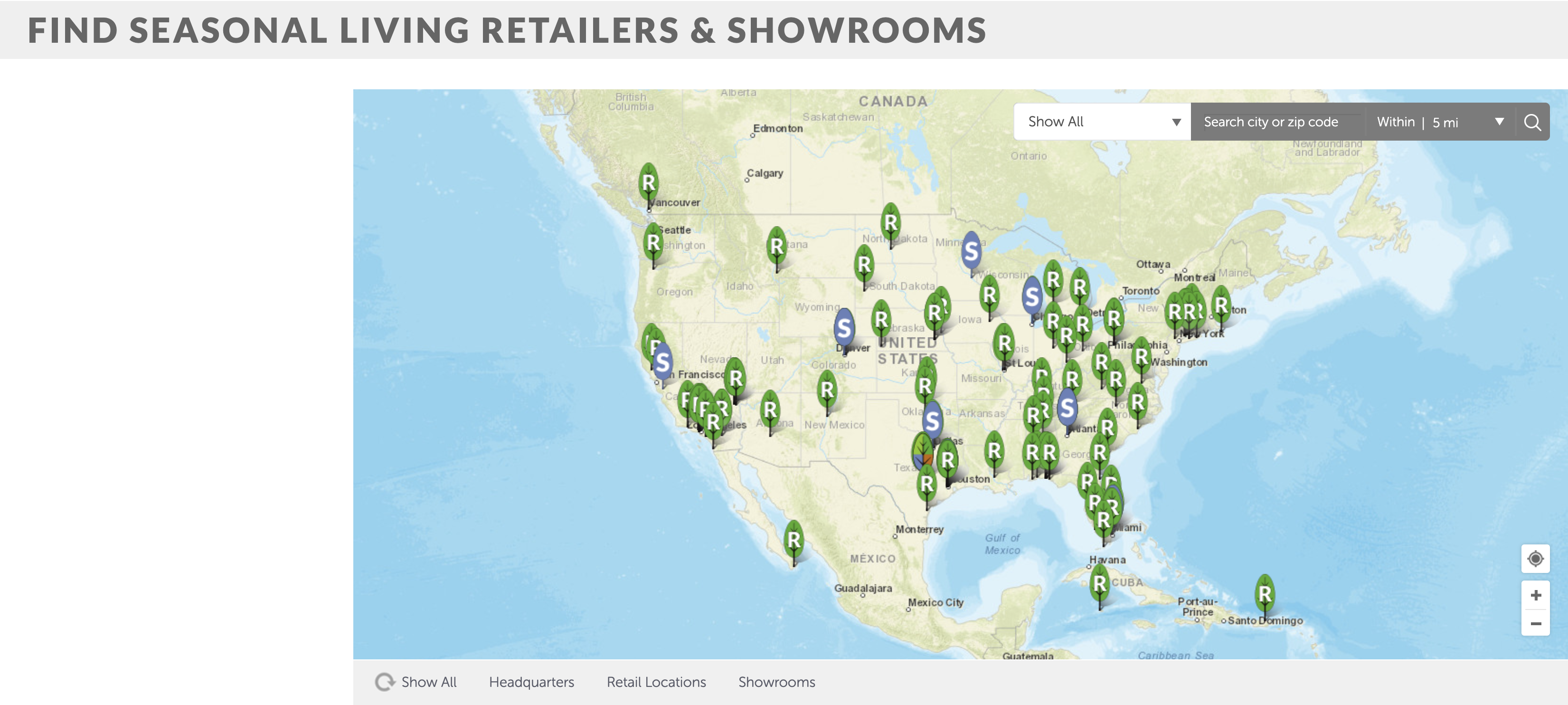**Caption:**

A detailed screenshot from a desktop website highlights the feature "Find Seasonal Living, Retailers, and Showrooms" located in the top left corner. The expansive layout, unsuitable for a mobile device, includes a drop-down menu with an option to "Show All." Users can search for locations by entering a city or ZIP code, with the ability to adjust the search radius from 5 to 50 miles. Below the search bar, there are options to "Show All," represented by a circular arrow, as well as categories labeled "Headquarters," "Retail Locations," and "Showrooms."

The main section of the image prominently features a detailed map of North America, pinpointing various showroom locations. Each type of location is marked distinctly: a green leaf with a white 'R' for retail stores, a purplish leaf or feather with a white 'S' for showrooms, and a unique multicolored leaf with shades of green, purple, and red standing alone.

The majority of the marked locations are concentrated on the East Coast of the United States, with a scattering across the central region from North Dakota to Texas, and notable clusters in Canada and the West Coast, particularly California and Seattle. The map also displays a few international locations, including spots in Mexico and Cuba. Overall, the map provides a comprehensive view of the business's various locations.